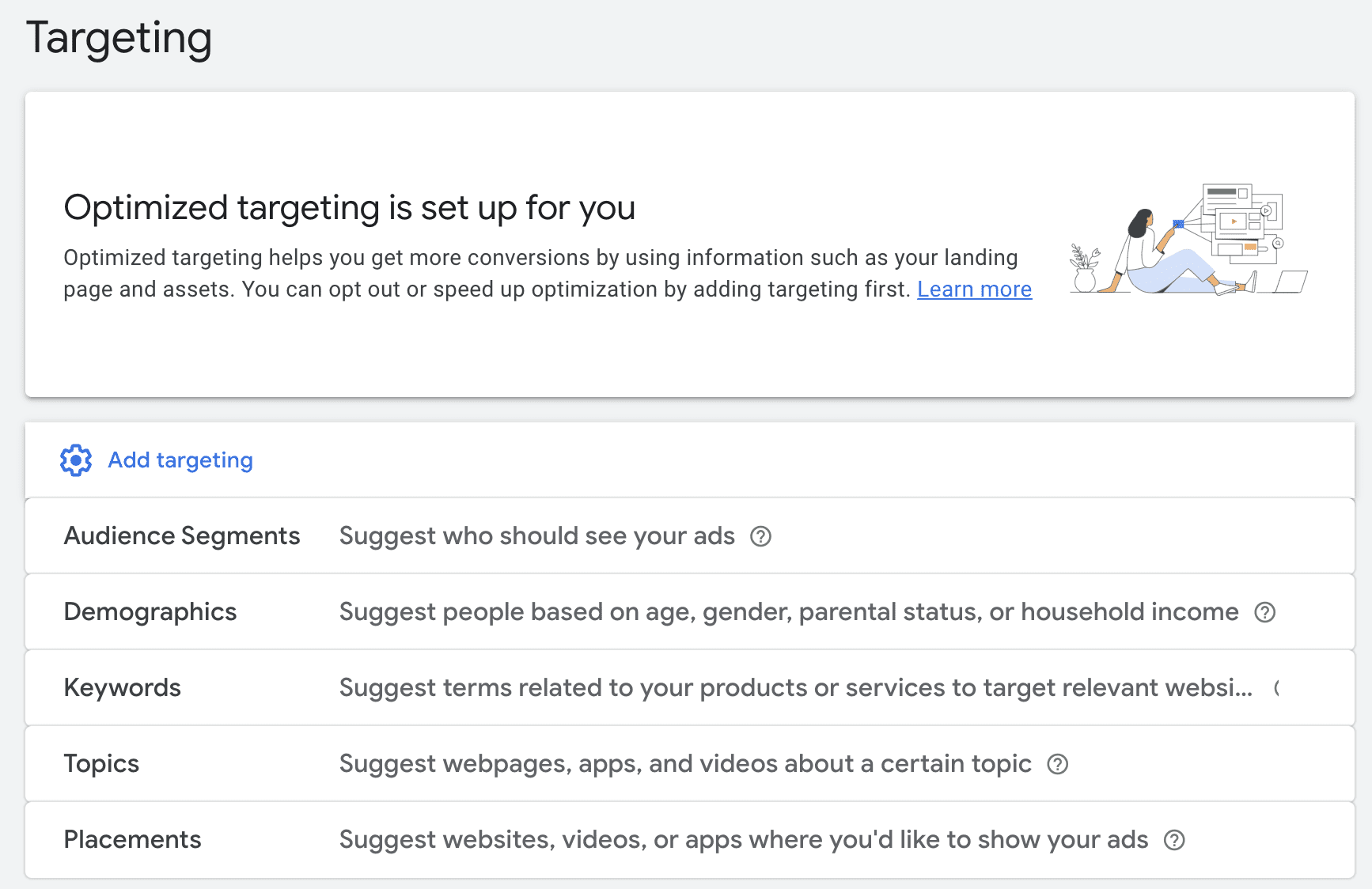The image has an off-white background with a bold black heading that reads "Targeting" in the upper left corner. Below that is a crisp, white, rectangular horizontal section with black lettering at the top reading, "Optimized Targeting is set up for you." Underneath, in smaller text, it explains, "Optimized Targeting helps you get more conversations by using information such as your landing page and assets. You can opt out or speed up optimization by adding Targeting first." Following this is a clickable "Learn More" link in a bright blue color, underlined.

To the right of this section, there is an animated illustration of a woman, seen from behind, facing something on the wall. Her feet are positioned towards the right edge of the image, and there is an indeterminate object behind her.

Below this, the off-white background continues and features a second vertical rectangular section. At the top left of this section is a Settings logo in the same bright blue, next to the text "Add Targeting," also in blue. Down the left side, the text "Audience Segments" is displayed, followed by "Suggest Who Should See Your Ads?" with a circled question mark beside it. Underneath, the term "Demographics" is printed, suggesting people based on "age, gender, parental status, or household income," with another circled question mark. The next line says "Keywords," indicating terms related to your products or services to target relevant websites, although the word gets cut off at the right edge. Further down, "Topics" suggests webpages, apps, and videos about a certain topic, again with a circled question mark. Finally, "Placements" advises on websites, videos, or apps where you'd like to show your ads, marked with another circled question mark. Thin, faint gray lines separate each section for clarity.